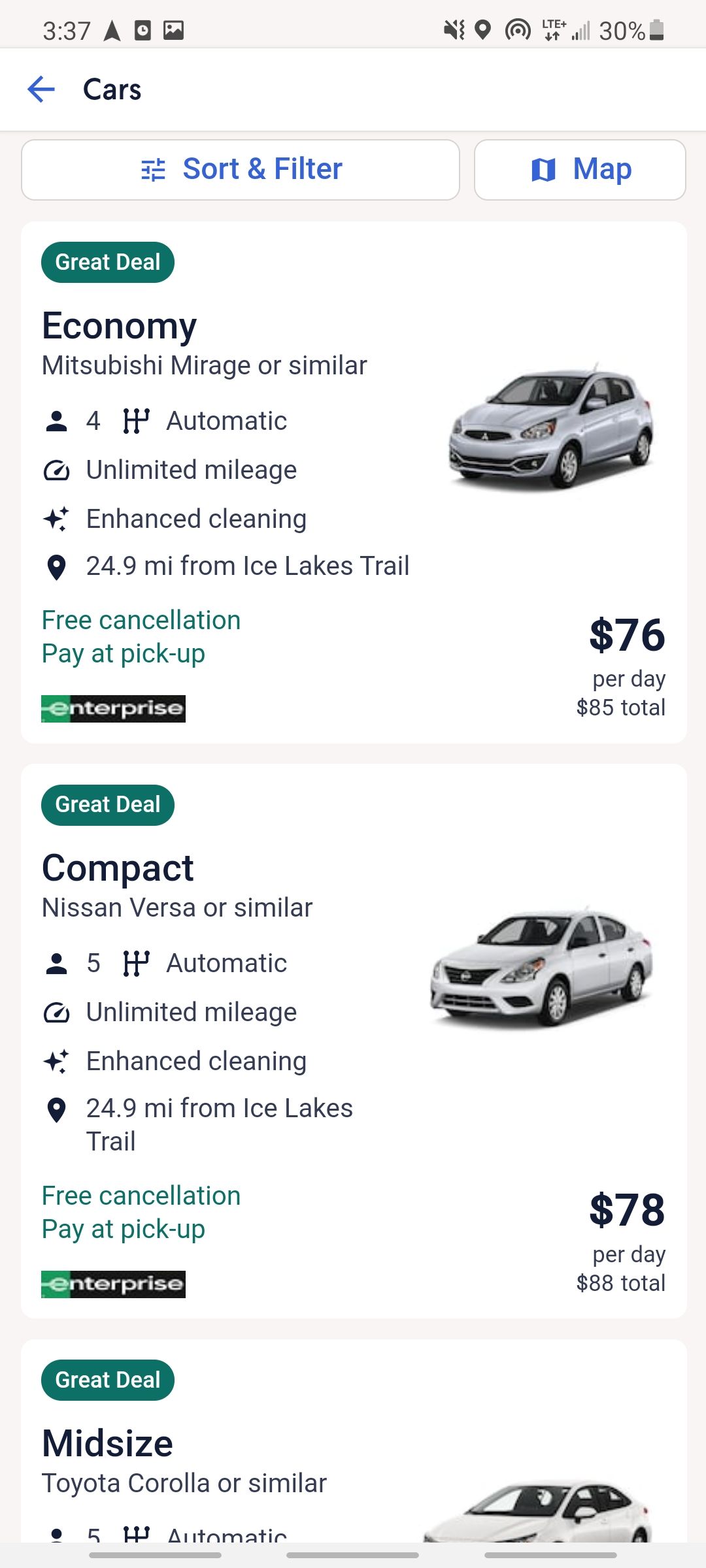Here's a cleaned-up and detailed caption for the image:

---

Screenshot of a Vehicle Rental App Interface

This is a detailed screenshot taken from a cell phone of an app interface used for renting vehicles. At the top of the screen, within a white bar with black text, the title "Cars" is displayed alongside a left-pointing blue arrow, indicating a back navigation option. Below this, there are two interactive buttons: "Sort and Filter" on the left side and "Map" on the right side. The "Sort and Filter" button allows users to filter available cars based on preferences such as type and price, while the "Map" button shows the locations where these cars can be picked up.

The main section of the screenshot displays three vehicle listings, each with a white background and a green bar marked "Great Deal" in white lettering.

1. **First Listing**: 
    - **Category**: Economy
    - **Model**: Mitsubishi Mirage or similar
    - **Price**: $76 per day, $85 total
    - **Additional Info**: Free cancellation, pay at pickup
    - **Location**: Specified
2. **Second Listing**:
    - **Category**: Compact
    - **Model**: Nissan Versa or similar
    - **Price**: $78 per day, $88 total
    - **Additional Info**: Unlimited mileage, enhanced cleaning
    - **Location**: Specified
3. **Third Listing**:
    - **Category**: Midsize
    - **Model**: Toyota Corolla or similar
    - **Details Visible**: Top portion of the listing only; visible text includes "five automatic," with the rest cut off by the screenshot.

The image captures the essential elements of the app, providing a glimpse into the options and features available to users looking to rent a vehicle.